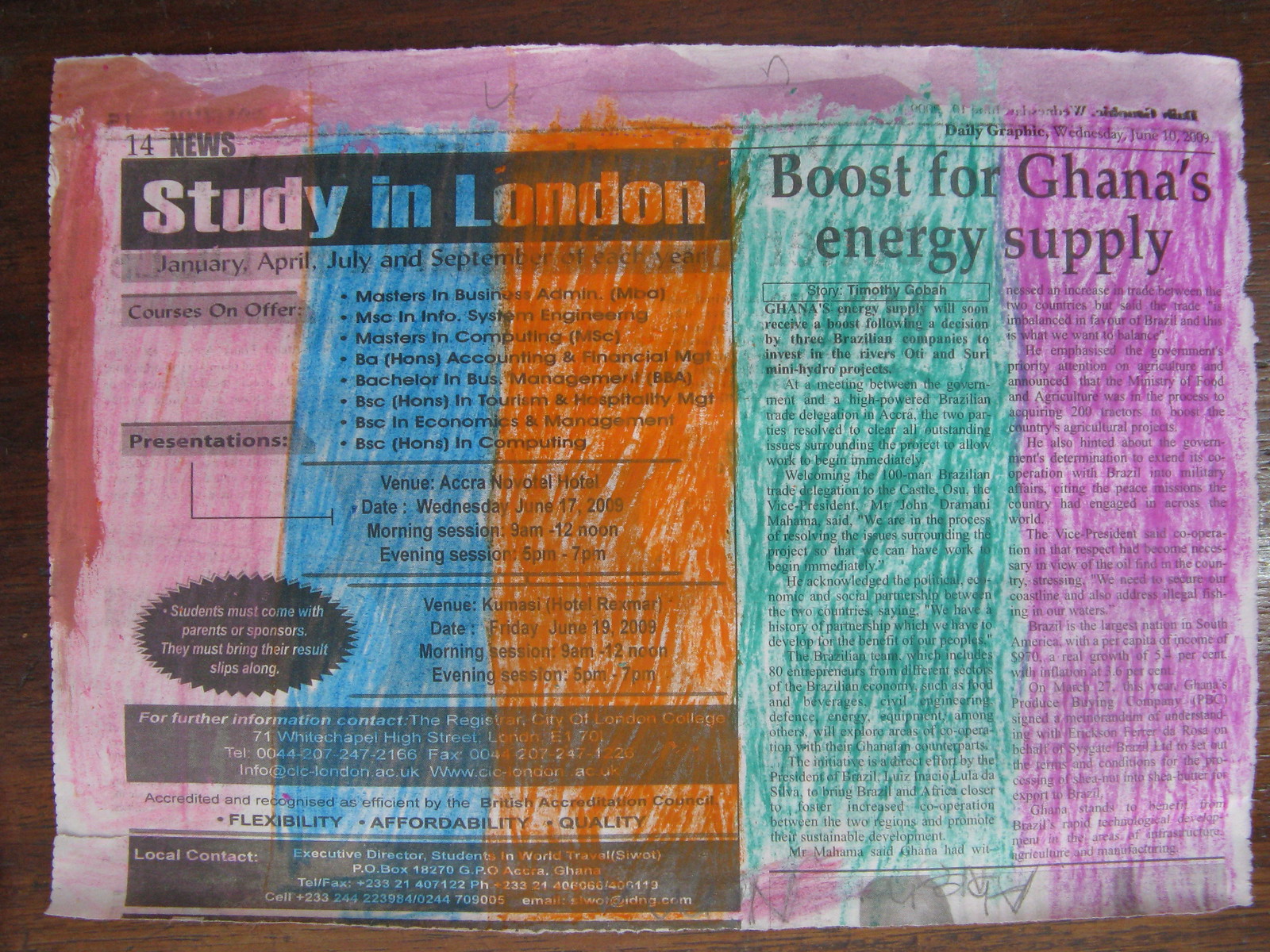This photograph depicts a torn rectangular newspaper clipping lying on a dark brown wooden table, positioned closer to the right and bottom edges of the image. The jagged edges of the newspaper suggest it has been ripped out. The top portion of the page has been colored in purple, and the rest of the clipping is divided into five vertical columns, each colored with crayons in distinct hues: pink, bright blue, orange, turquoise, and purple from left to right. In the pink, blue, and orange columns at the top, black rectangles with the white text "Study in London" are featured, while the turquoise and purple columns display the headline "Boost for Ghana's Energy Supply." The text "14 News, Study in London, January, April, July, and September of each year" is visible on the left side of the image, corresponding to the pink and blue columns. The crayon coloring gives the impression that a child may have used the newspaper as a drawing surface, further enhanced by the bright and cheerful color choices.